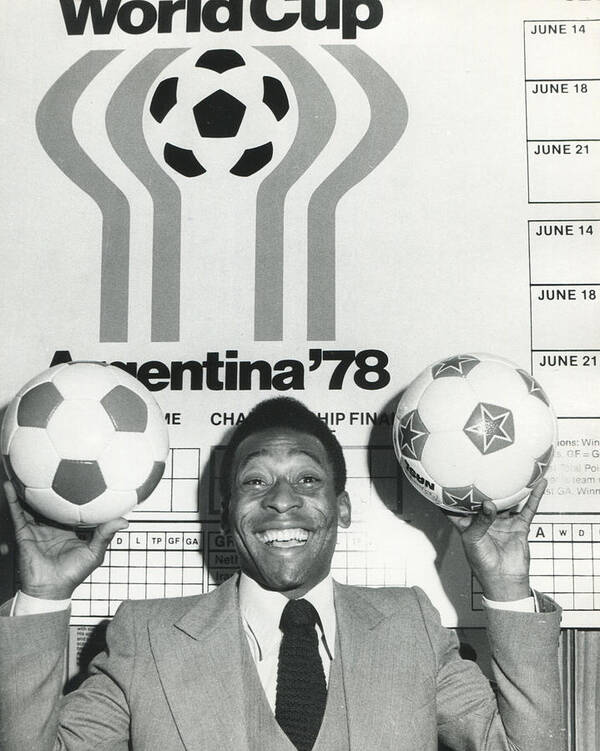This black and white photograph captures the legendary soccer player Pele, a black man with a radiant smile, dressed in a sophisticated suit comprising a gray jacket, a white shirt, and a dark knit tie. He stands prominently at the front bottom of the image, proudly holding up two soccer balls—one with a traditional honeycomb pattern in his left hand and a distinct one featuring stars in his right. Behind him, a poster reads "World Cup Argentina 78" and includes a small soccer ball emblem surrounded by gray streaks. To the right of the image, a list of dates is visible in brackets, detailing June 14th, June 18th, and June 21st, suggesting the timing of significant events or matches, possibly related to the championship final as indicated by the placard.